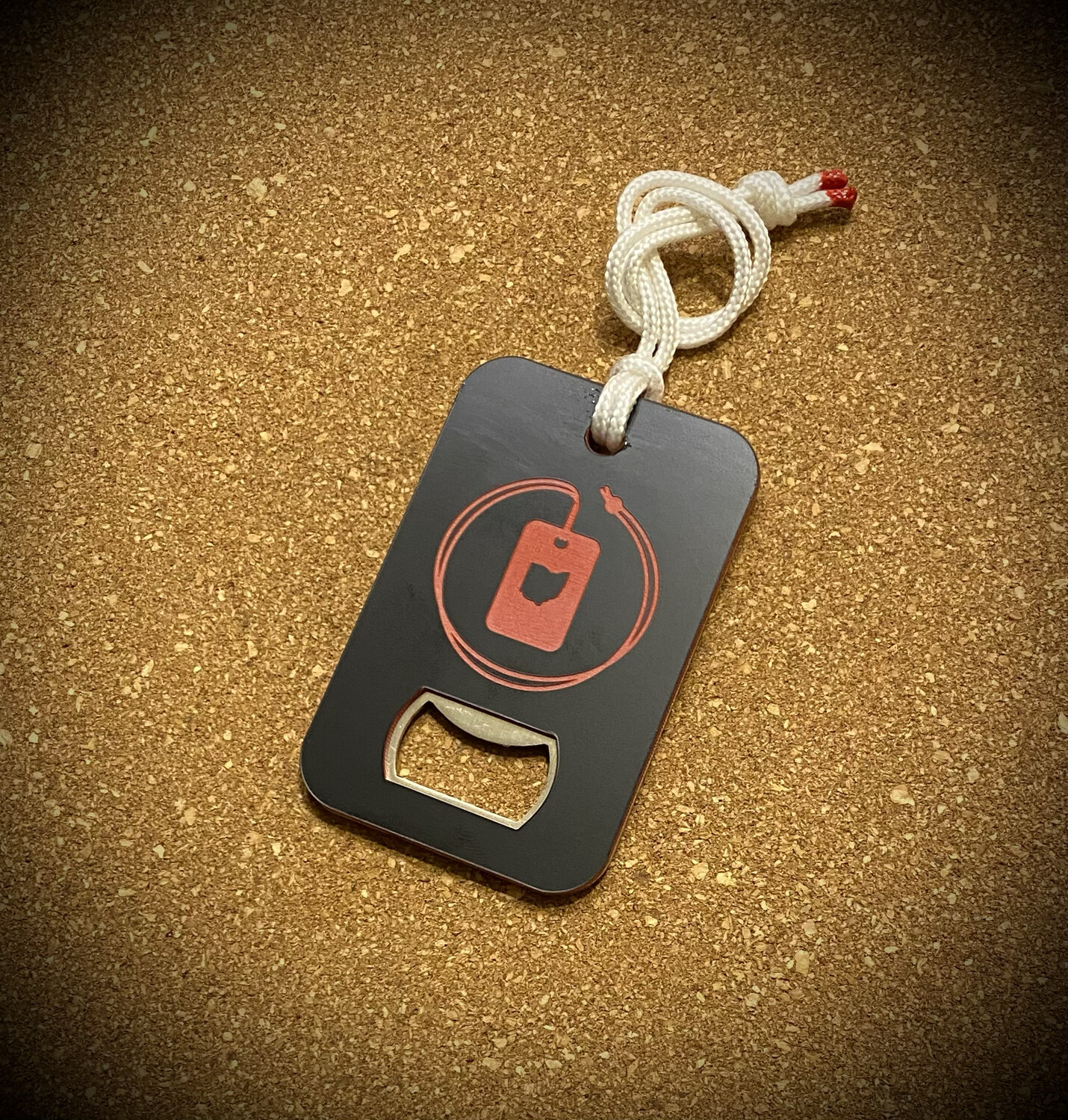The photograph is a vertically rectangular, full-color image taken indoors under artificial lighting, without a border. The corners of the image are darkened, almost black, creating a vignette effect, while the primary background consists of a brown, stony, compacted sand-like surface. 

At the center of the image is a black card resembling a credit card or a piece of cardboard. This card features a central design consisting of a red rectangle with looping red wires that nearly form a complete circle. The lower section of the card includes a rectangular cutout with rounded edges, serving as a functional bottle opener. This opening is lined with metal, and one of the lips is pronounced, presumably to facilitate bottle opening.

Extending from a hole at the top of the card is a thin white rope, tied in a knot, which loops through a hole. The rope has red tips, adding a touch of color contrast. The overall appearance of the object, coupled with its setting on the brown, pebbly background, gives the image a distinct, tactile quality.